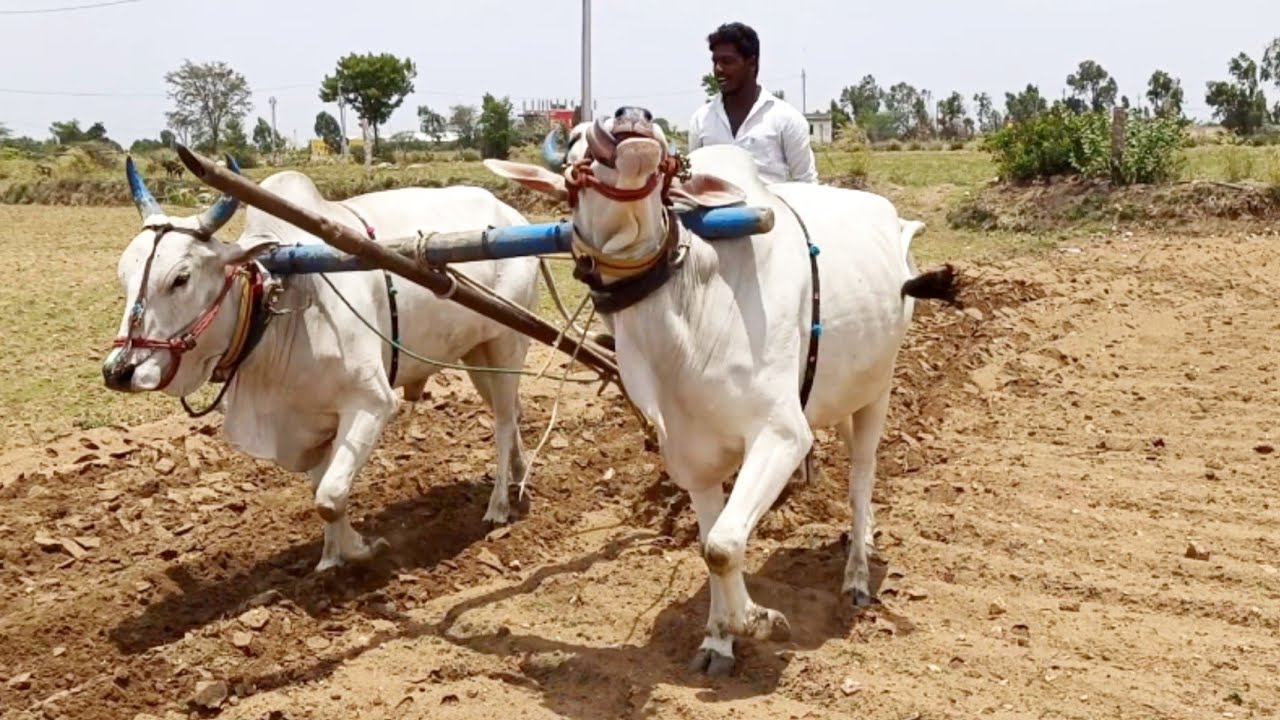In this outdoor scene, two white oxen with distinctive blue horns and saggy necks are harnessed together, connected by a wooden yoke and straps around their necks. They are plowing a field of dry, brown soil. One of the oxen has a browner face, giving it a unique appearance. Behind them stands a dark-skinned Indian man wearing a white button-down shirt. He guides the oxen as they work, using a bamboo log attached between them to till the soil. The background features a pale, partly gray sky, green-leaved trees, and bushes, with patches of wild grass and a farm field.